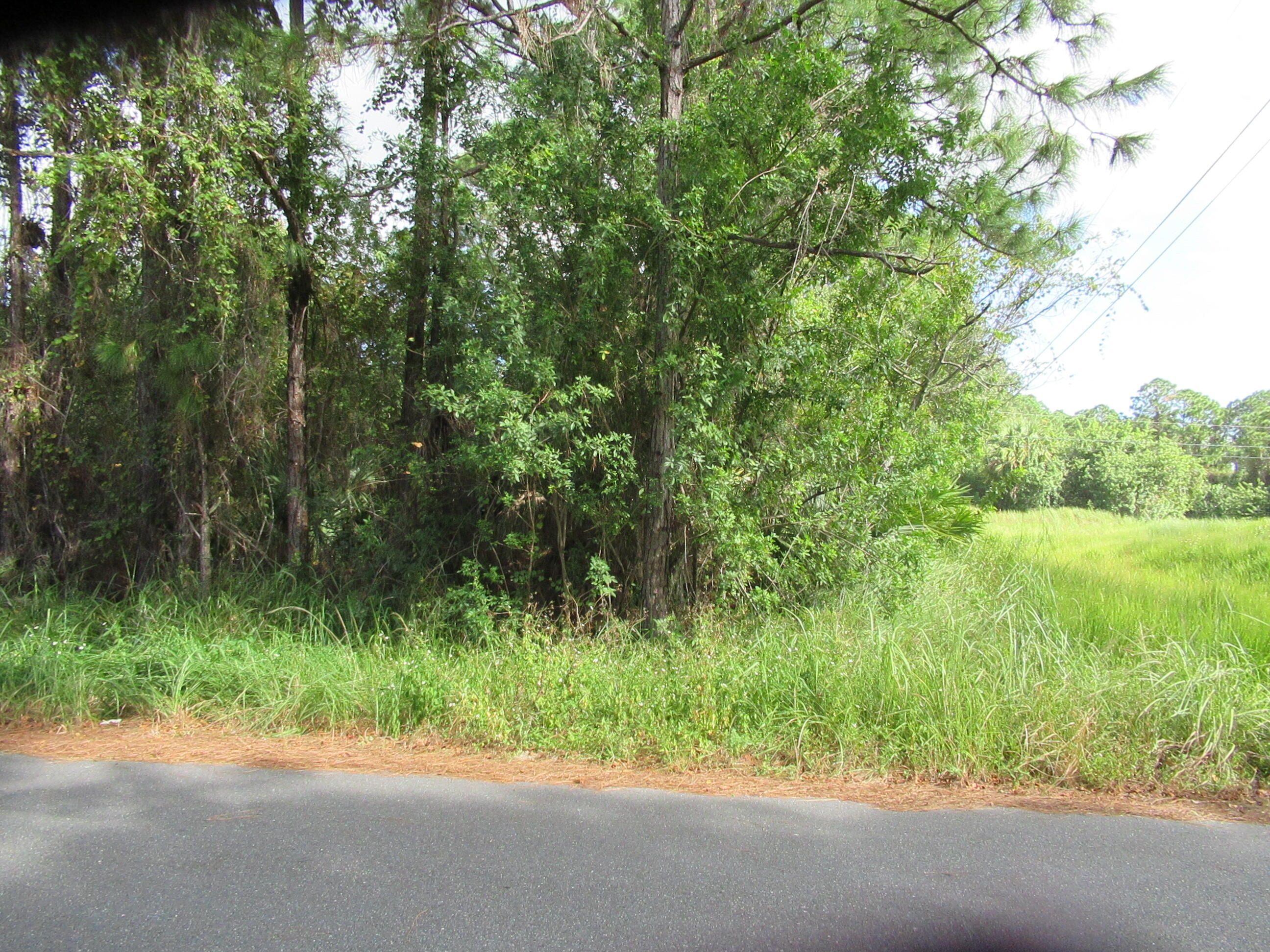The photograph captures the edge of a dense forest at the end of a residential cul-de-sac. In the foreground, a concrete road gives way to a stretch of dead grasses and unkempt, long green grass. Just beyond the road, a lush expanse of verdant grasses and varied foliate begins, interspersed with numerous slender, brown bark-covered tree trunks. These trees are tall and dense, displaying a thick canopy of green leaves that partially hides the sky. The tree line weaves into the background, creating a sense of depth as it snakes into the distance. To the right side of the image, a wide, grassy field extends, covered in thick, green blades that contrast with the more structured residential street. This rich natural scene, with its combination of wild, flourishing greenery and the clear demarcation of the forest edge, evokes a serene border between cultivated land and untouched nature.